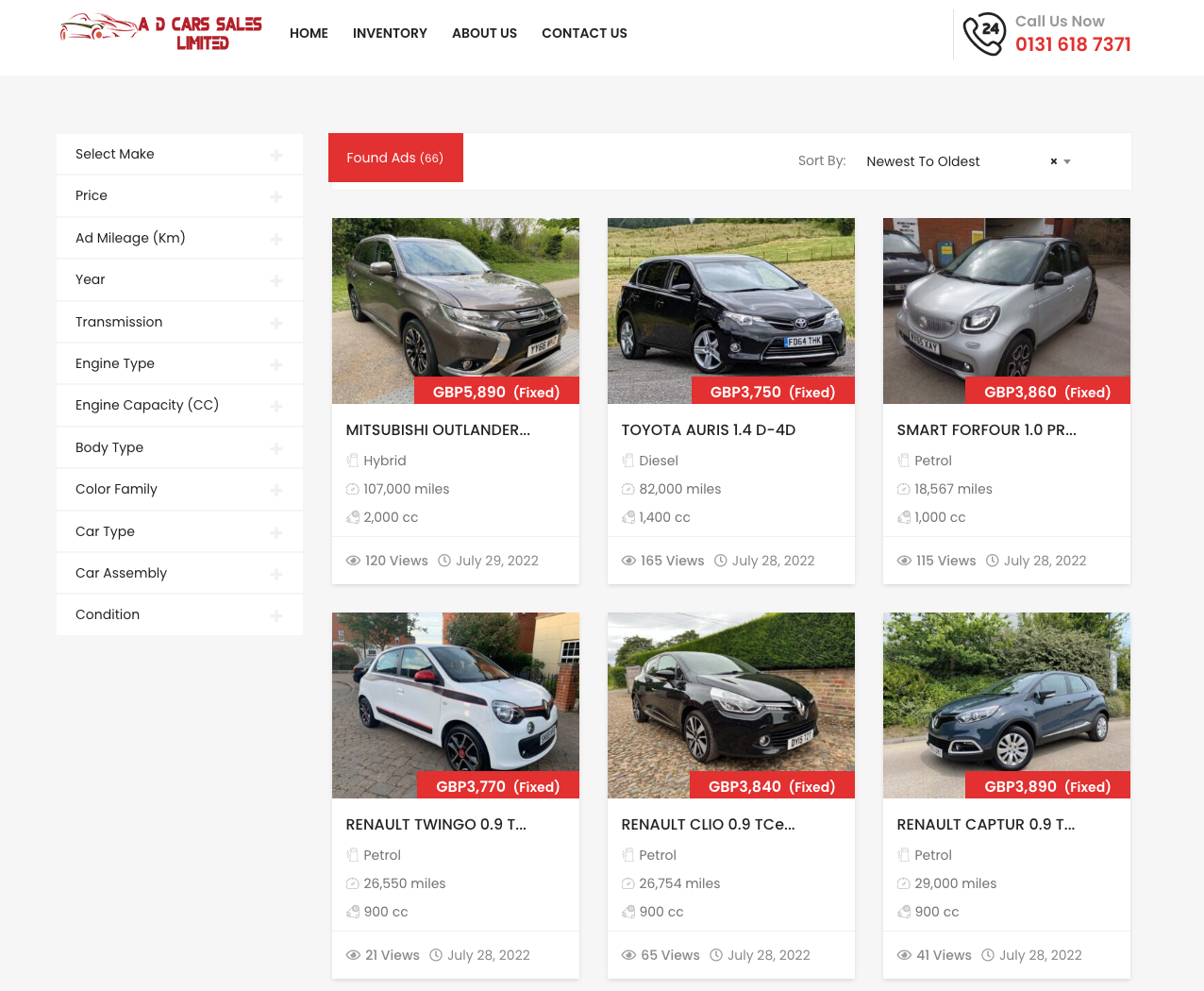Screen capture of a website named "AD Cars Sales Limited," an online platform for purchasing cars. The website features a navigation menu at the top with tabs labeled "Home," "Inventory," "About Us," and "Contact Us." It also prominently displays a 24-hour contact number for customer inquiries. 

On the left side of the screen, there is a detailed search filter panel that allows users to refine their car search based on the following criteria: make, price, mileage in kilometers, year, transmission type, engine type, engine capacity in cubic centimeters (cc), body type, color, family, car type, car assembly, and condition.

The main section of the screen displays a list of six cars, each with an accompanying photograph. The listed vehicles include:
1. Mitsubishi Outlander
2. Toyota Ilaris L4D4D
3. Smart 4.4 1.0 PR
4. Renault Twingo 0.9
5. Renault Clio 0.9
6. Renault Captur 0.9

Each car listing provides essential information, making it easier for potential buyers to compare and make informed decisions.